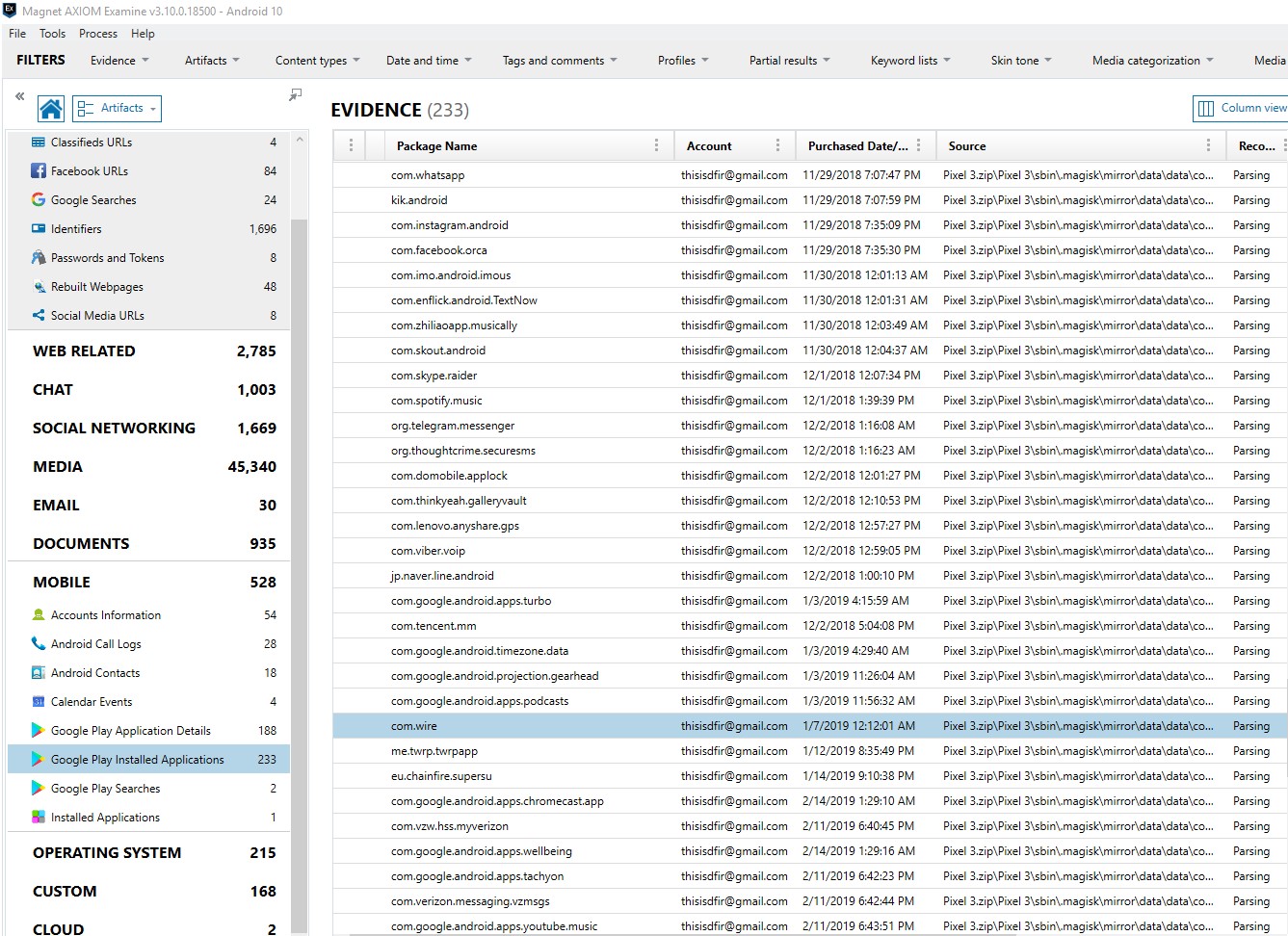This image appears to be a detailed screenshot of a software interface, likely for a forensic or data analysis tool. 

The screenshot itself is landscape-oriented, approximately square in shape, and features a thin white border along the top. At the top-left corner of this border is a black shield-like logo next to text reading "Magnet AXIOM Examine Version 3.1.0.18500 Android 10."

Directly below this is a long gray toolbar containing several menu options: File, Drop-down menu, Tools, Process, and Help. Beneath this, another black header bar includes filter and sort options, such as Evidence, Artifacts, Content Types, Date and Time, Tags and Comments, Profile, Partial Results, Keyword Lists, Skin Tones, Media Categories, and more.

On the left side of the interface, there is a vertical column with a blue icon resembling a house, alongside several categorized pop-up menus. These categories include Classified URLs, Facebook URLs, Google, and other sections that classify information into Web-Related, Chat, Social Networking, Media, Email, Documents, Mobile and Operating System, Custom, and Cloud categories.

To the right of this side column is a larger white box titled "Evidence," displaying a count of 233. This section is organized into columns labeled Package Name, Account, Purchase Date, Source, and Recon. The files listed here appear complex and lengthy, potentially containing coded information that might require specialized knowledge to interpret fully.